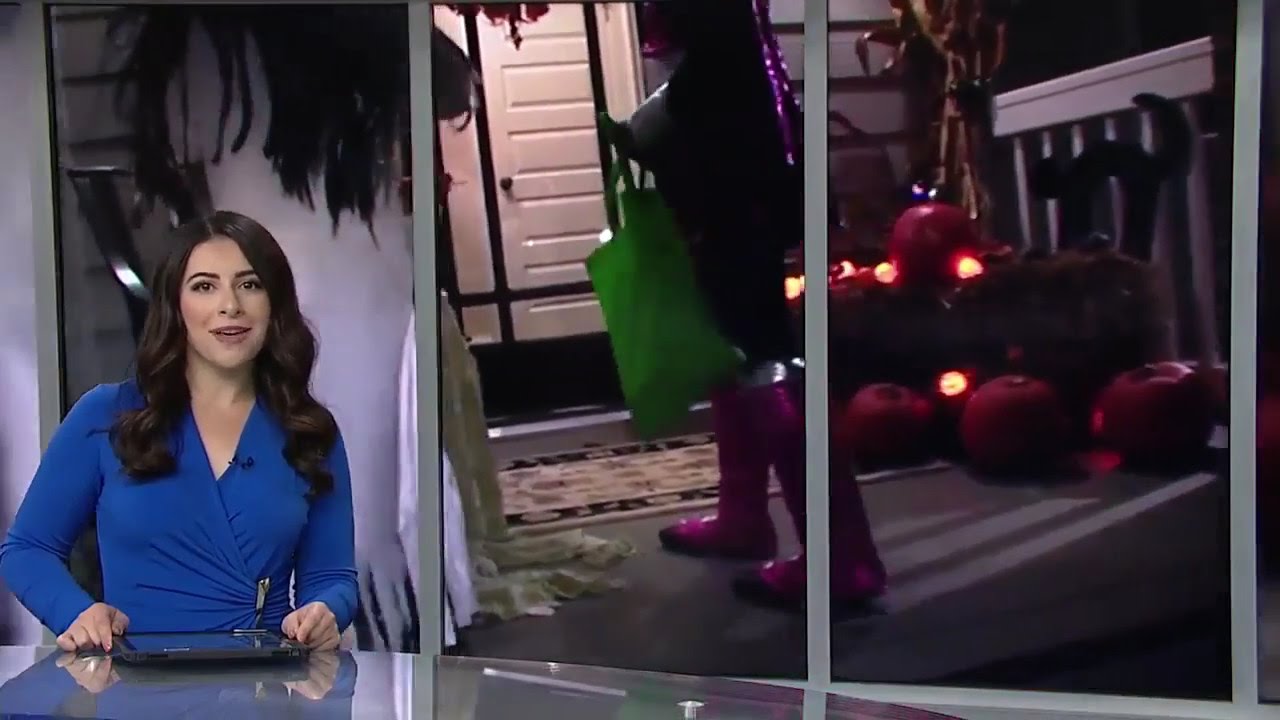In the image, a news presenter with long dark brown hair, styled over her right shoulder, is seen sitting at a modern glass desk. She is donning a blue, long-sleeved wrap dress with a V-neck, and there is a small microphone clipped to her dress. An iPad lays on the table in front of her, and she is looking directly at the camera with her hands resting on the device. Positioned on the left side of the frame, she appears poised and professional, with a neatly made-up face.

Behind her, a large screen spans the background, displaying a vivid Halloween scene. This backdrop features a child, seen from the rear and somewhat indistinct due to the darkness, ascending a set of steps adorned with lit pumpkins. The child, seemingly dressed for trick-or-treating, is wearing pink rain boots and holding a green bag, likely for collecting candy. The porch scene they are walking towards includes a welcome mat and a white door, with a glimpse of a white railing. Various Halloween colors—blue, tan, black, orange, yellow, green, purple, pink, and white—create a festive atmosphere, reinforcing the theme of the news segment, which likely revolves around Halloween activities, costumes, and trick-or-treating preparations.